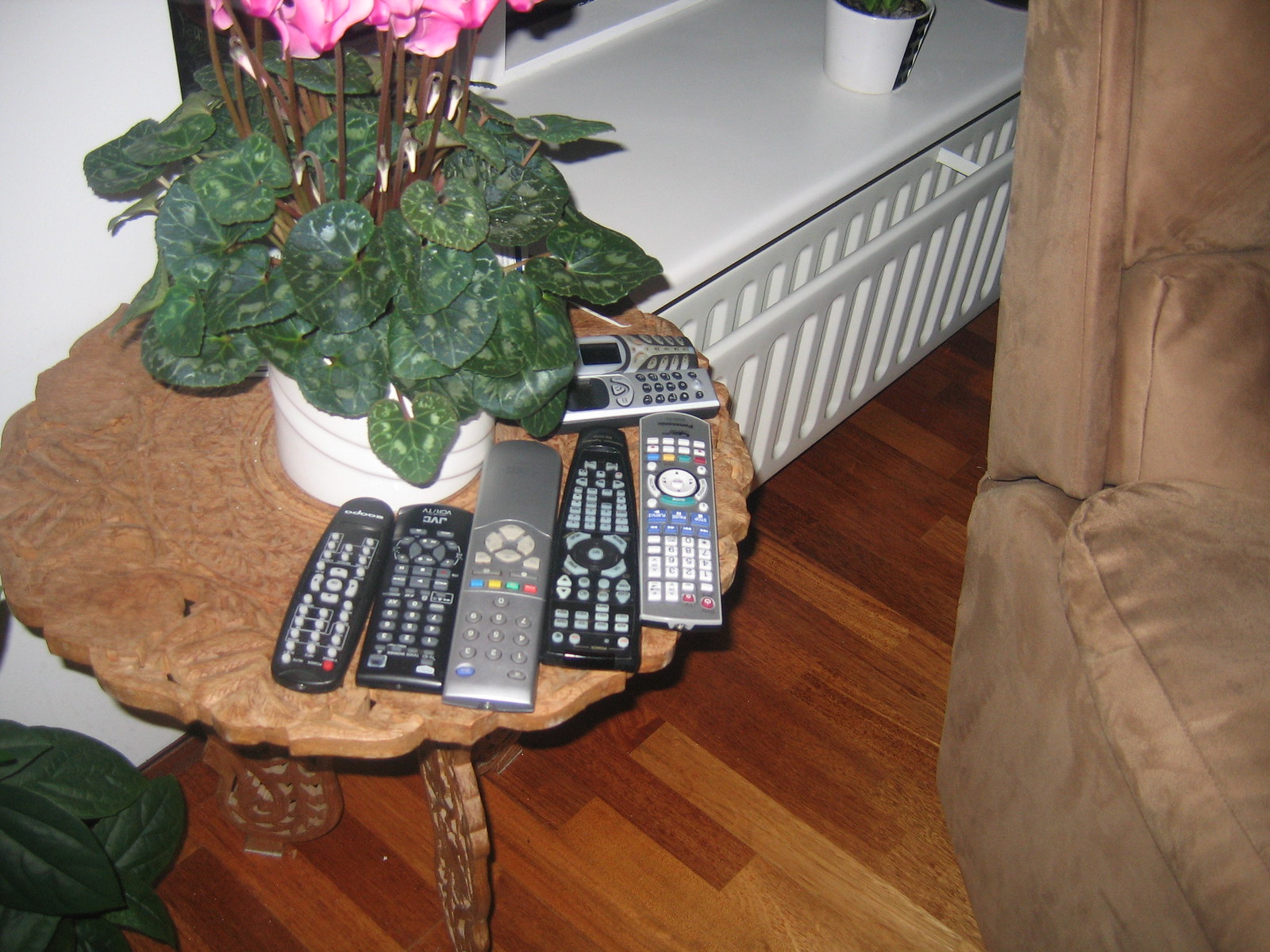In this detailed photograph, the main subject is a round wooden table with a scalloped, flower-like edge and ornately carved legs. The table, situated on a diagonally aligned medium-brown wooden plank floor, hosts an array of items. There are five remote controls fanned out towards the front: three black, one gray with a light gray outline, and one silver with black trim. These remotes feature colorful buttons in red, green, yellow, and blue. To the right side of the remotes, two early 2000s-style mobile phones with small, square screens and physical buttons are placed. At the center of the table, a white flower pot with two brown decorative lines holds a plant with large green, slightly pointed leaves. Brown stems extend to reveal pink flowers just creeping into the frame. The background includes a black window, suggesting the photo may have been taken at night, and a white radiator running underneath the windowsill. Positioned towards the upper middle of the windowsill is a small white container. In the bottom left corner of the image, a piece of dark green crumpled fabric is visible. To the right of the table, a medium-brown chair or couch upholstered in plush fabric is partially in frame.